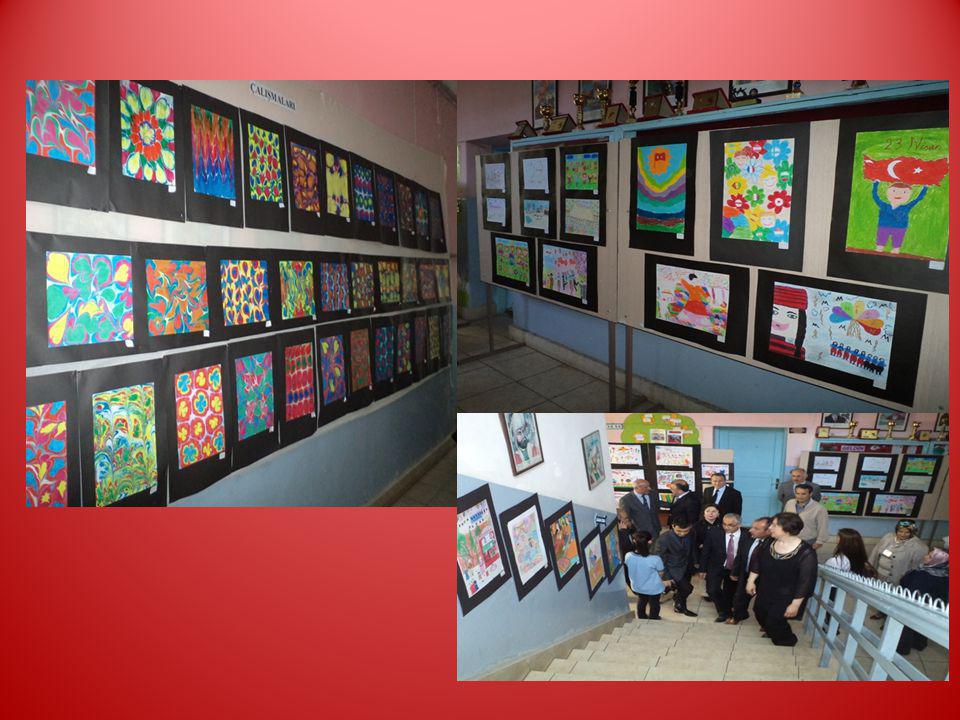The image displays a vibrant school art gallery set against a red background, showcasing a collage of two overlapping photographs. In the left photo, three rows of children's artwork are lined up, each piece featuring abstract shapes in vivid colors like yellow, red, and green, all set against black backgrounds. The right photo extends this display with more rows of similarly framed artwork, but also includes a distinct piece showing a boy in a blue long-sleeve shirt and purple shorts, holding a red flag with a white moon and star, against a dark green background. Below this, there’s a scene of adults, dressed professionally, ascending stairs adorned with more colorful artwork. Their presence is captured as if by a security camera, emphasizing their movement towards the gallery. The tiled floor and blue and white walls frame this collection, making it clear that it’s an elementary school art show, teeming with creativity and community engagement.